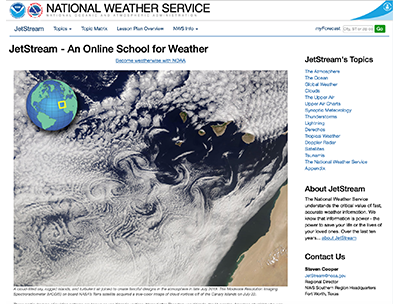This image is a screenshot of the National Weather Service's website. At the top, the header reads "National Weather Service." Below it, there is smaller text that appears to mention "Jetstream," which is described as "an online school for weather." The main section of the page prominently features a weather map displaying snowy conditions, with a visual depiction of snow that appears whitish and watery. To the side, there is a section labeled "Jetstream Topics," followed by a list of various topics. Below this, another section is titled "About Jetstream," accompanied by a paragraph of text. The bottom of the page contains a "Contact Us" link. Due to the small font size, the finer details are difficult to discern.